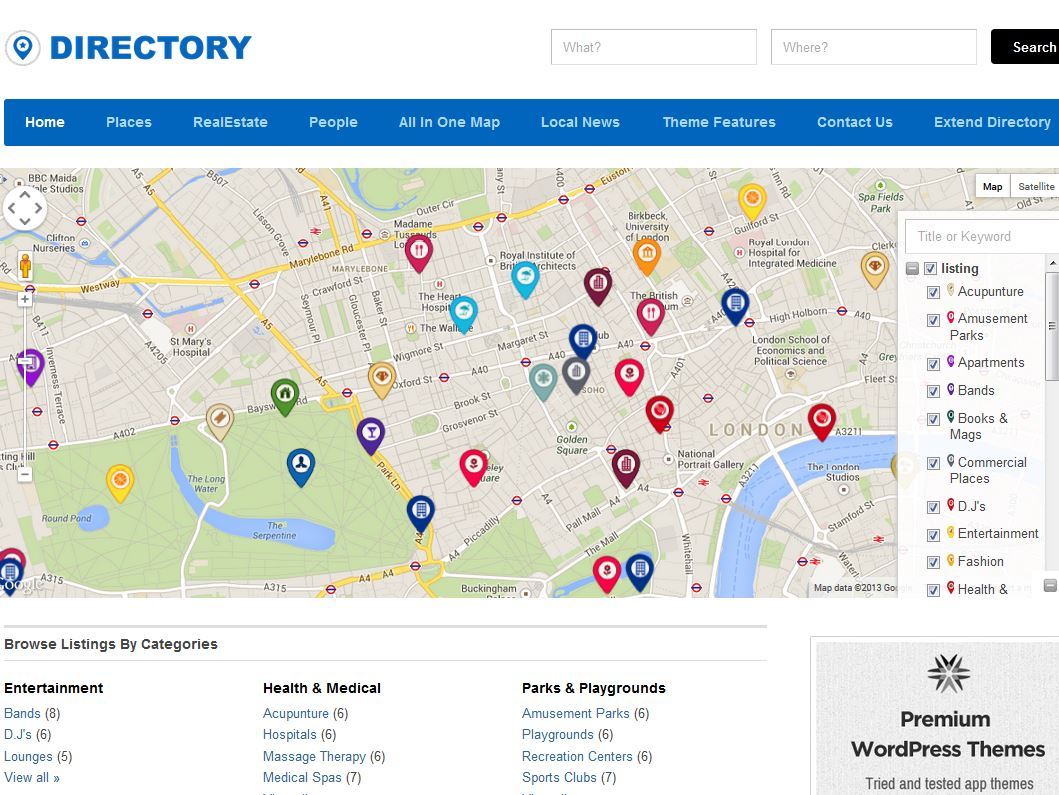The image depicts an application interface organized around a directory. The top left corner prominently displays the title "DIRECTORY" in large blue capital letters. Occupying the top right corner are two editable fields designed for inputting search criteria: one for what you're searching for, and the other for where you're searching. Adjacent to these fields is a black search button.

Below the search area, a blue horizontal banner spans the entire width of the screen, containing navigation headings. These headings include HOME, PLACES, REAL ESTATE, PEOPLE, ALL IN ONE MAP, LOCAL NEWS, THEME FEATURES, CONTACT US, and EXTEND DIRECTORY. The HOME section is currently highlighted, appearing slightly folded and white.

Dominating the main area of the screen is an extensive map adorned with various colored markers in blue, yellow, pink, red, and more. This map allows users to visualize different locations. To the right of the map is a keyword chart featuring checkboxes that enable users to choose which markers to display. For instance, selecting the "fashion retailers" checkbox highlights them with yellow markers. Other options include markers for apartments, amusement parks, and additional amenities, each with corresponding colors.

Beneath the map and keyword chart are several category listings, each representing different types of locations such as entertainment venues, health and medical facilities, and parks and playgrounds. Users can click on these categories to explore further.